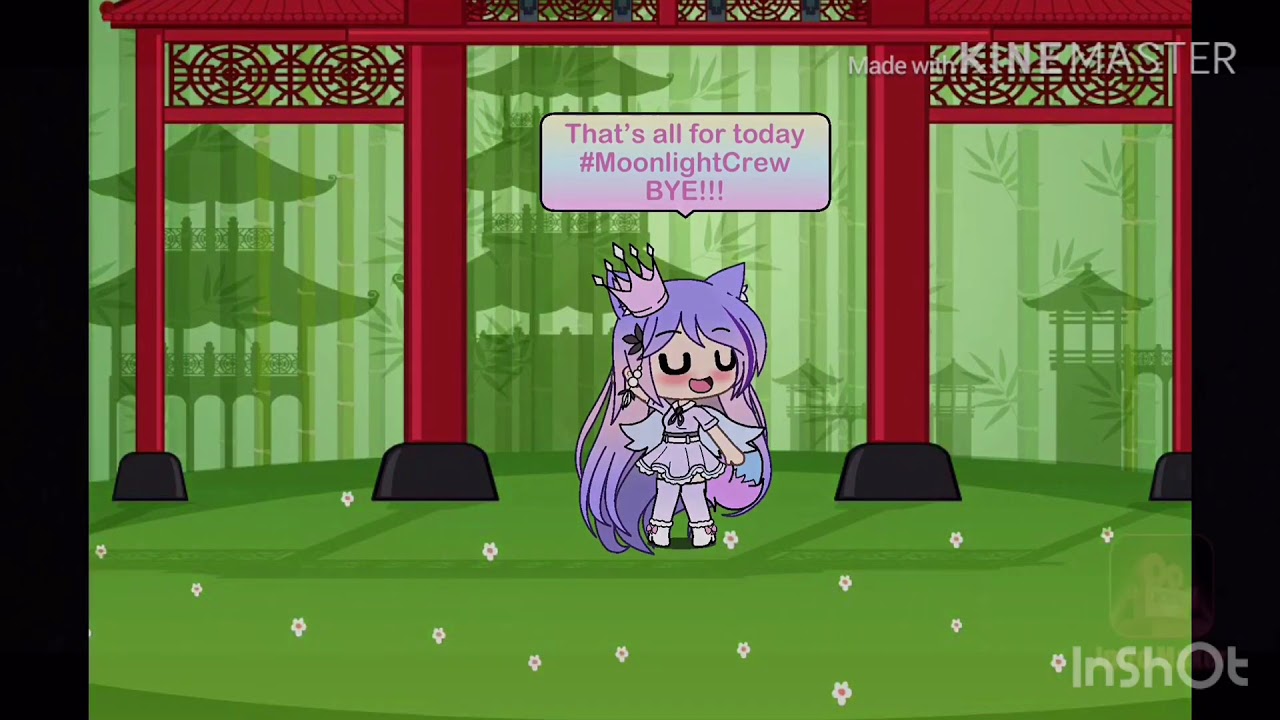In the center of this vibrant digital image is a chibi-style anime character, appearing as a young princess or queen. She has floor-length, flowing purple hair adorned with a light pink crown and purple cat ears. Her delicate, light skin features rosy cheeks, closed eyes shaped like the letter 'U', and an open mouth as if she is joyfully speaking. She is waving with her left hand while her right arm rests by her side. The girl is dressed in a cute, light purple dress paired with high-heeled boots with ribbons, and she has dusky gray wings extending from her back. 

She stands on a lush green field dotted with white daisy flowers, with a red, square archway (torii gate) rising above her and Asian-inspired buildings silhouetted in the background. Above her head is a speech bubble reading, "That's all for today. #MoonlightCrew, bye!" with three exclamation points. The image features a diverse palette of colors including green, black, white, orange, pink, purple, blue, dark red, and gray. In the bottom right corner, it reads "inShot," and in the top right, it says "Made with Kinemaster." This meticulously crafted image captures a whimsical and playful atmosphere, perfectly illustrating the charming character at its center.